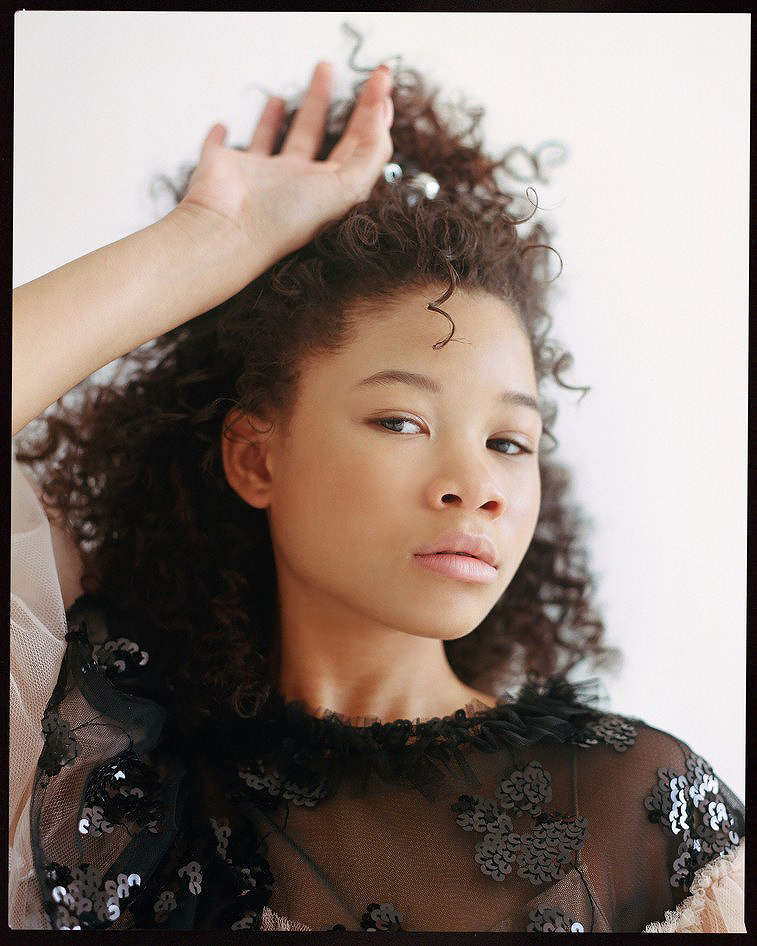This color portrait photograph captures a young African-American woman, likely in her teens, set against a white studio background. She has light skin and clear complexion, highlighted by minimal makeup. Her hair, meticulously styled into elegant, non-frizzy ringlets, is adorned with pearls and gathered up on top of her head. She poses with a model-like grace, her right hand bent at the elbow with the back of her hand resting atop her head. Her expression is neutral, perhaps slightly melancholic, as she looks down towards the viewer.

She is dressed in a sheer black blouse featuring a ruffled neck and decorated with black sequin flowers, creating a sophisticated and textured look. The garment transitions into a mesh ballet pink fabric just below the ruffled neck, adding a delicate contrast. This carefully composed image, full of intricate details, exudes a sense of artistic realism and representationalism.